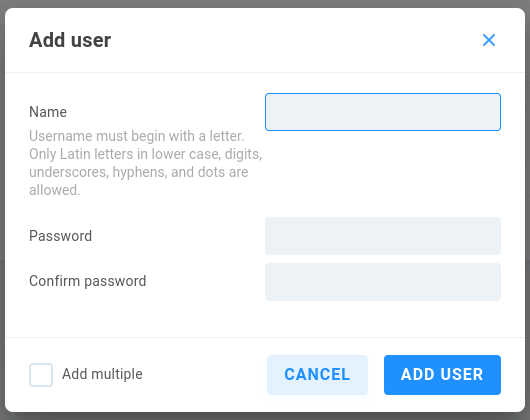The image depicts a user interface pop-up window for adding a user on a website's control panel. The pop-up title, "Add User," is prominently displayed in the upper left corner. Opposite this, in the upper right, a blue "X" is present to close the window. Below the title, on the left side, is a labeled field "Name" accompanied by guidelines: the username must begin with a letter and can include lowercase Latin letters, digits, underscores, hyphens, and dots. A form field to the right allows the input of the username.

Further down, aligned to the left, are the labels "Password" and "Confirm Password," each paired with a corresponding form field on the right for entering and confirming the password, respectively. In the lower left corner of the pop-up, there's an unchecked checkbox labeled "Add Multiple." On the lower right, two buttons are visible: a light blue "Cancel" button with blue text and a blue "Add User" button with white text. The overall layout is designed for user-friendly navigation to facilitate adding new users through this pop-up interface.